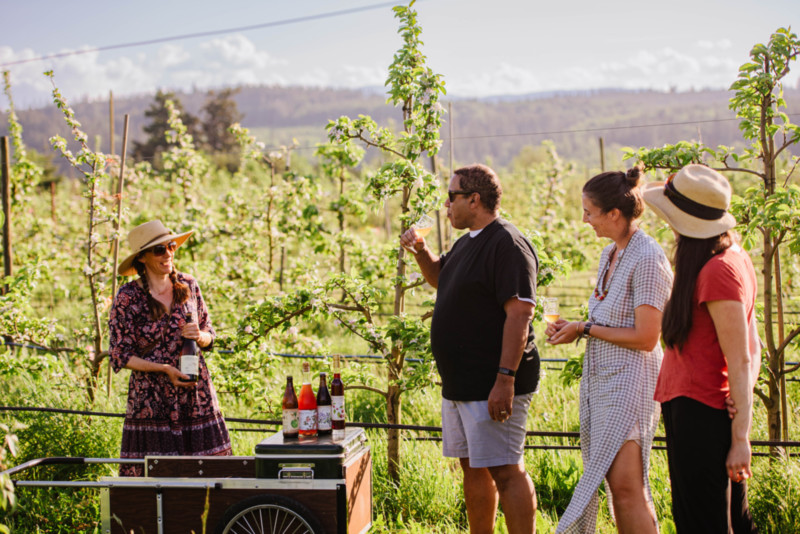In this detailed outdoor image, four people stand beside a small, mobile beverage cart, which appears to be part of a vineyard tour. The cart, which has two wheels and a horizontal handle, serves as a concession stand and holds a cooler topped with four bottled beverages of various colors. The woman managing the stand wears a wide-brimmed straw hat, dark sunglasses, and a burgundy-colored, pink-and-black speckled sundress. She is holding one of the bottles.

Three customers, all wearing sunglasses, stand in front of the cart. The first is a slightly overweight man dressed in light shorts and a dark shirt, sipping from a drink. The second person is a woman with her hair in a bun, wearing a light cotton checkered dress, smiling as she holds a glass of wine. The third customer is another woman in a red shirt, dark pants, and a straw hat decorated with a black bow. 

The background reveals a picturesque vineyard setting with rows of green plants, possibly grapevines, supported by cables. In the distance, slightly hazy hills and scattered trees are visible under a sky with some clouds. The overall scene suggests a serene day in the countryside, capturing a moment of leisure and enjoyment.